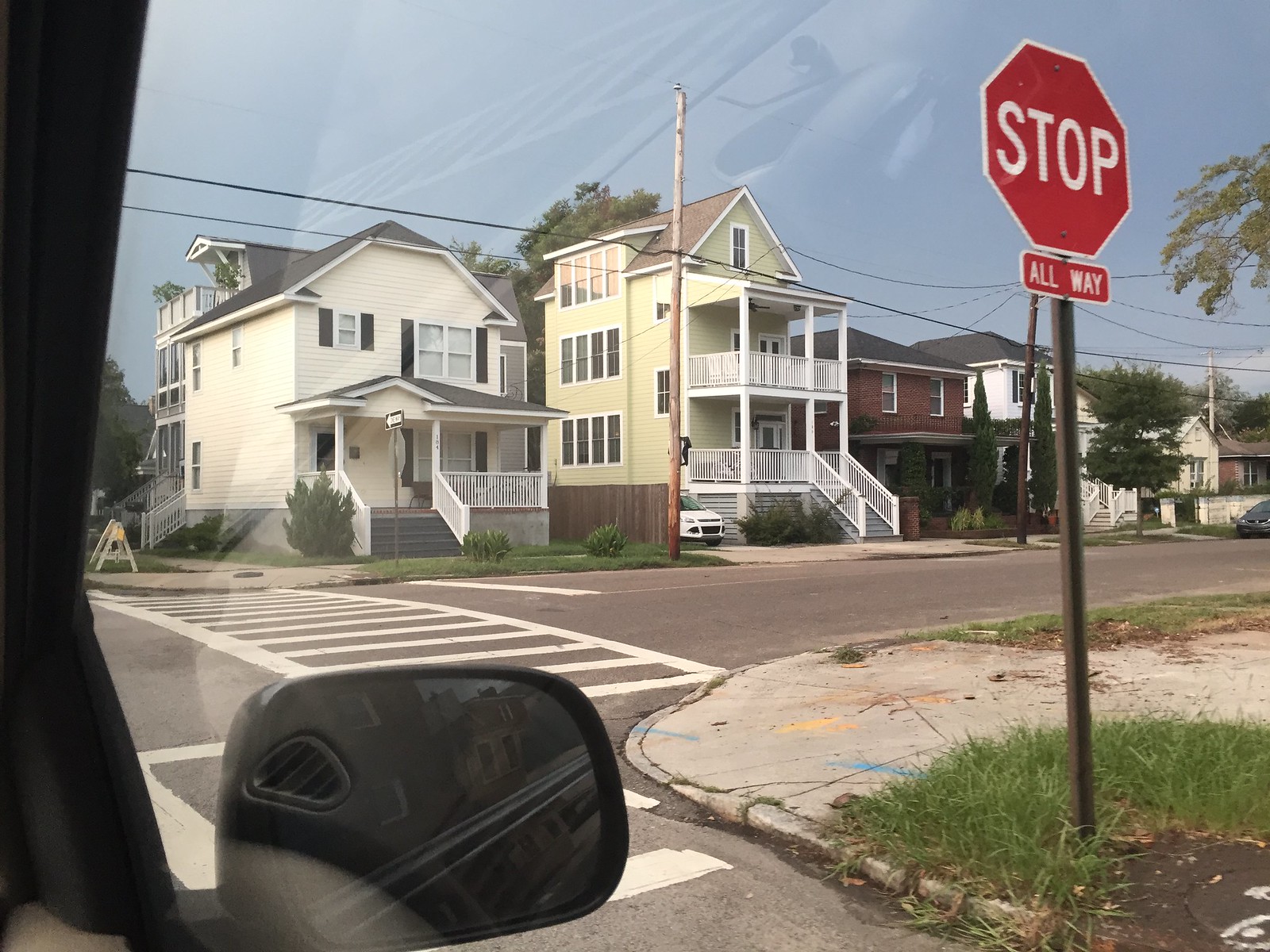This image captures a street scene from the perspective of someone inside a car looking out the passenger side window. In the lower left-hand corner, part of the car's black frame and side mirror are visible, along with a bit of reflection on the glass. The car is stopped at a corner, evidenced by the prominent stop sign surrounded by a small patch of grass. The sidewalk beneath the stop sign has patches of dirt, and there is painted pavement indicating a pedestrian crossing.

Across the street, a collection of multi-storied houses in different colors are arranged neatly along the corner. On the far left, there is a white house, followed by a tall, light yellow house with a two-story deck porch and a tan roof. Next comes a red brick house. Off to the right of these, additional houses can be seen, including one with cream walls and black shutters. The sky is an almost clear blue with minimal cloud coverage, though there appears to be some reflection from the car window creating light etching effects in the sky.